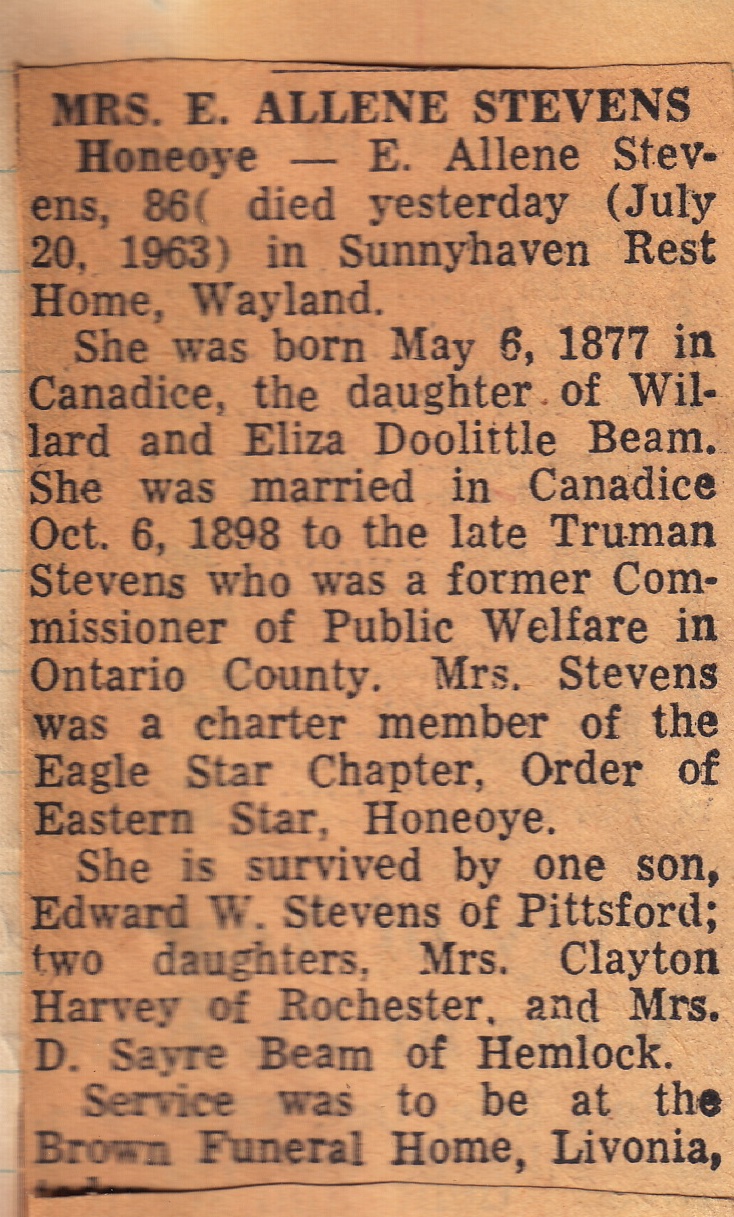This is a close-up image of a yellowed and slightly orange-tinted newspaper cut-out, indicating its age. The clipping features an obituary for Mrs. E. Allen (Elaine) Stevens, who passed away on July 20th, 1963, at the age of 86 in Sunny Haven Rest Home, Wayland. Mrs. Stevens was born on May 6, 1877, in Kandis, to Willard and Eliza Doolittle Bean. She married the late Thurman Stevens in Kandis on October 6, 1898; he was a former Commissioner of Public Welfare in Ontario County. A charter member of the Eagle Star Chapter Order of the Eastern Star, Mrs. Stevens is survived by one son. The obituary, devoid of any photographs or drawings, includes additional information about her surviving family and details regarding her funeral services.